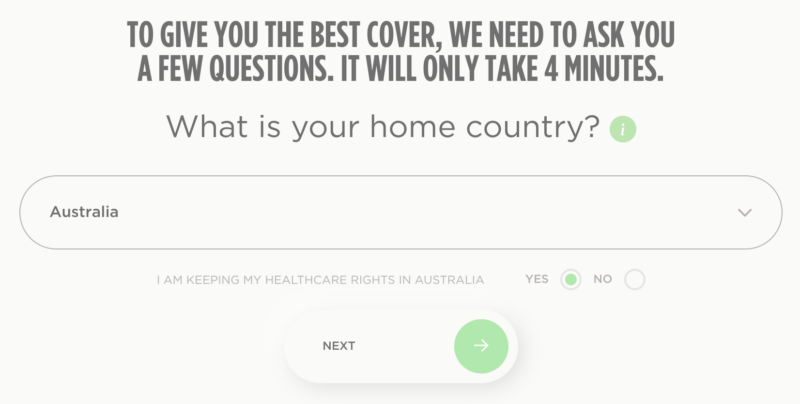The screenshot depicts a webpage designed to help users explore their health care options, specifically targeted towards residents of Australia. The interface begins with a prominent message in gray-black capital letters: "TO GIVE YOU THE BEST COVER, WE NEED TO ASK YOU A FEW QUESTIONS. IT WILL ONLY TAKE 4 MINUTES." The phrase "4 MINUTES" is uniquely written with the number "4."

Beneath this, the first question asks, "What is your home country?" accompanied by an information icon for additional guidance. A dropdown menu or list provides various countries, with "Australia" prominently selected in this instance.

Further down, there is a statement in gray text: "I AM KEEPING MY HEALTH CARE RIGHTS IN AUSTRALIA," followed by two options, "Yes" and "No," each accompanied by a circle. The selected option, indicated by a green highlight, is "Yes."

At the bottom of the screen, there is a green circular button with a right-pointing arrow, labeled "Next," allowing users to proceed to the following step.